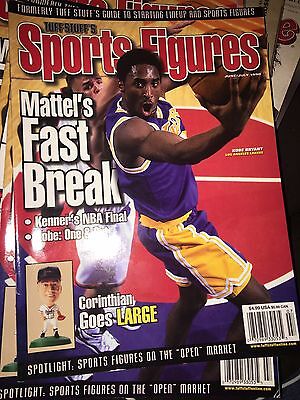This photograph is of a sports magazine cover titled *Sports Figures*, prominently displayed in red text with a white outline at the top. The main focus is on two black basketball players standing on a wooden basketball court. The player on the left is in a white jersey, while the player on the right wears a purple and yellow jersey. Above their heads, against a black background with barely legible white text, the headline reads, "Formerly Tough Stuff's Guide to Starting Lineup Red Sports Figures." To the left of the players, white text in varying sizes states, "Mattel's Fast Break Kenner's NBA Final." Below this is an inset image of a baseball figurine, next to which the white text reads, "Corinthian goes large," with the word "large" highlighted in yellow. At the bottom, in a black bar with white text, it reads, "Spotlight Sports Figures on the 'Open' Market." To the lower right is a white rectangle housing a black barcode and small black text for purchasing the magazine.